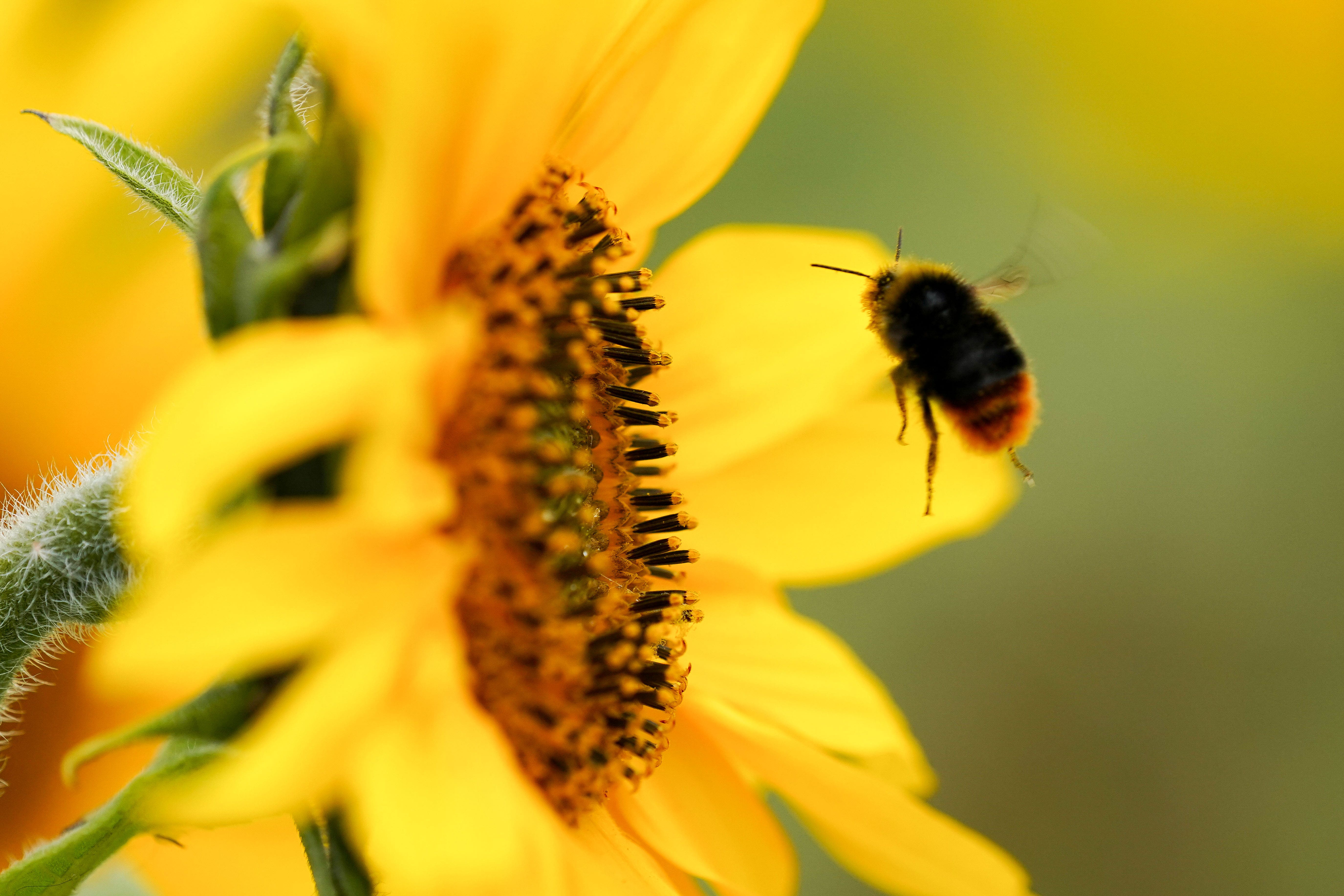This is a highly detailed, close-up photograph of a honeybee in mid-flight, approaching the vibrant yellow petals of a sunflower. The image showcases the bee from the back, revealing its yellow face, two antennae, and a black back with a light brown, slightly amber-tipped tail. The sunflower, also prominently featured, has a bright yellow center adorned with a multitude of short, peg-like black and yellow protrusions that resemble the teeth of a comb or brush. The flower's stem, visible on the left side of the image, has fine white hairs. In the background, the image transitions into a blurred mix of gray, light bluish-green, and forest green hues, providing a natural, earthy backdrop. The entire composition draws the viewer's focus to the intricate details of both the bee and the sunflower, creating a vivid, immersive scene.